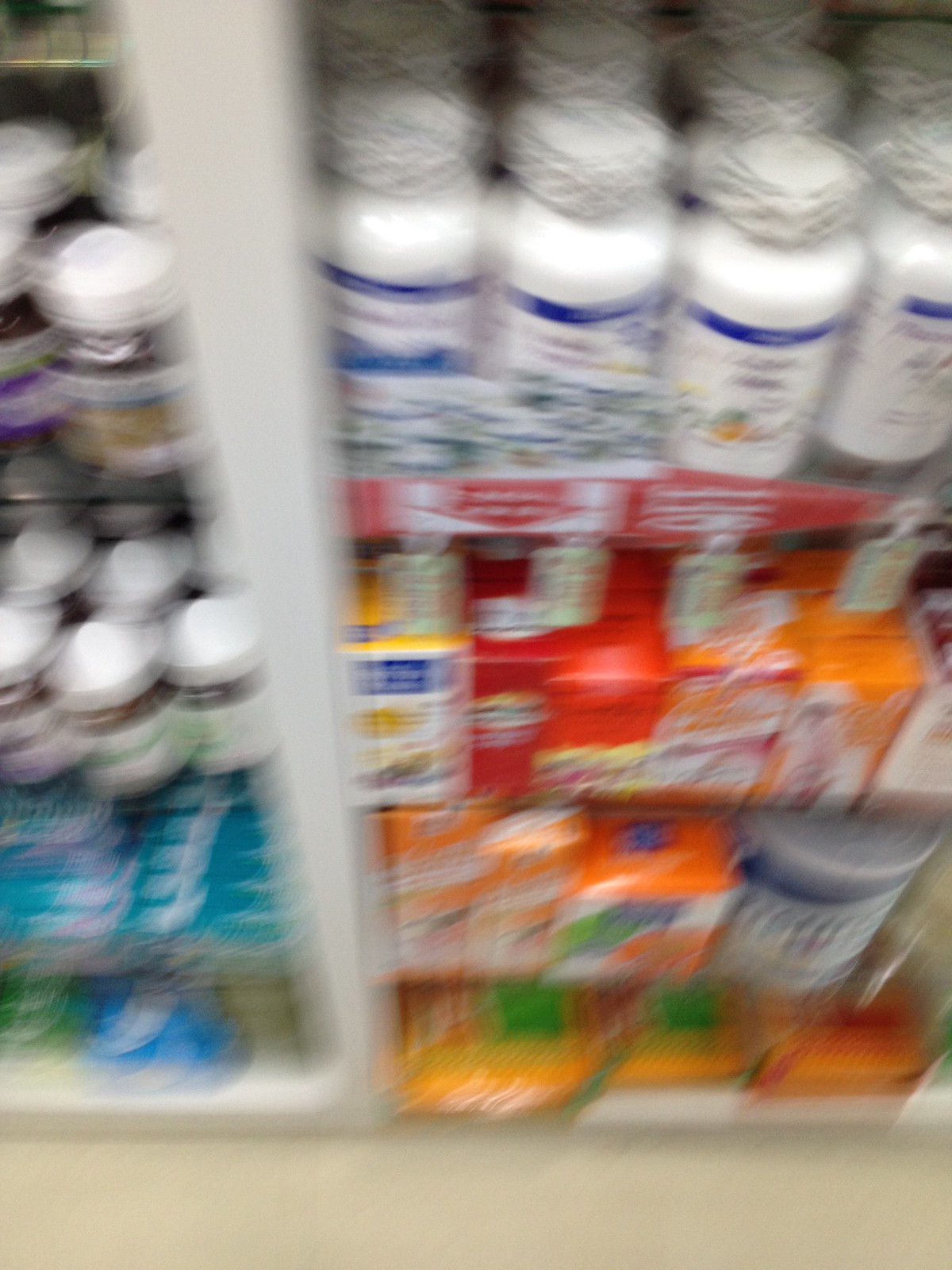The image depicts a somewhat blurry and out-of-focus photograph of what appears to be a pharmacy display shelf. The white shelves have glass planks inside and are divided by a white vertical bar that runs down about a third of the way. At the top right of the shelf, there are small white plastic pill containers. The two top left shelves feature various jars with white caps and colorful labels. Below these jars on three shelves, there are multiple boxes, with prominent colors being red, orange, yellow, and aqua. On the lower two left shelves, there are long-shaped and round boxes. There is a red banner running horizontally along one of the middle shelves, potentially serving to indicate pricing or product information. The detailed view of the containers reveals some with white caps that have safety writing around them. The overall impression is that of a blurred snapshot capturing the diverse array of products neatly arranged on the pharmacy shelves.